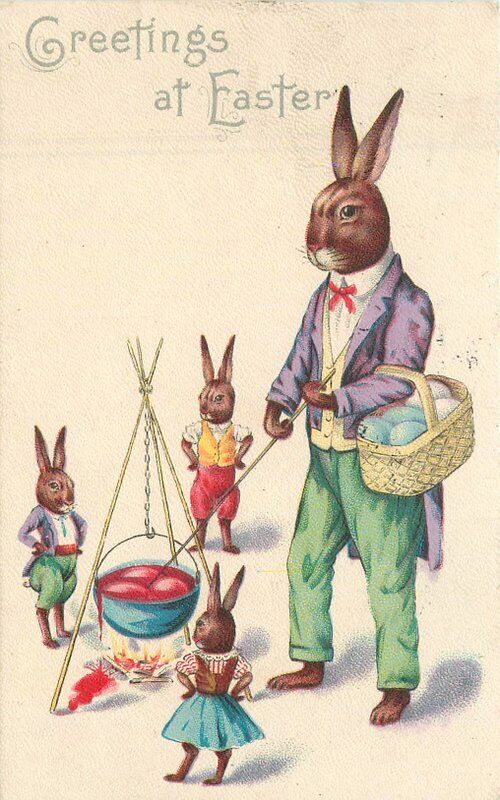The image depicts an old vintage Easter card in a portrait layout with a light pink background. In the upper left corner, the text "Greetings at Easter" is written in two lines of grey, creative fonts. On the right side stands a tall brown Easter bunny dressed in a white shirt, red bowtie, cream vest, and black jacket with tails, accompanied by green pants and bare feet. This sophisticated bunny holds a yellow basket filled with blue and white eggs over his left hand, while with his other hand, he manages a wire disappearing into a pot suspended over a flame with a red substance inside. Surrounding the main bunny are three smaller bunnies—two dressed in pants, vests, and jackets, and one female wearing a skirt—all brown and standing around the cooking area. The scene suggests the elder bunny is coloring eggs with his children, evident by the cozy arrangement around the fire and the communal activity.